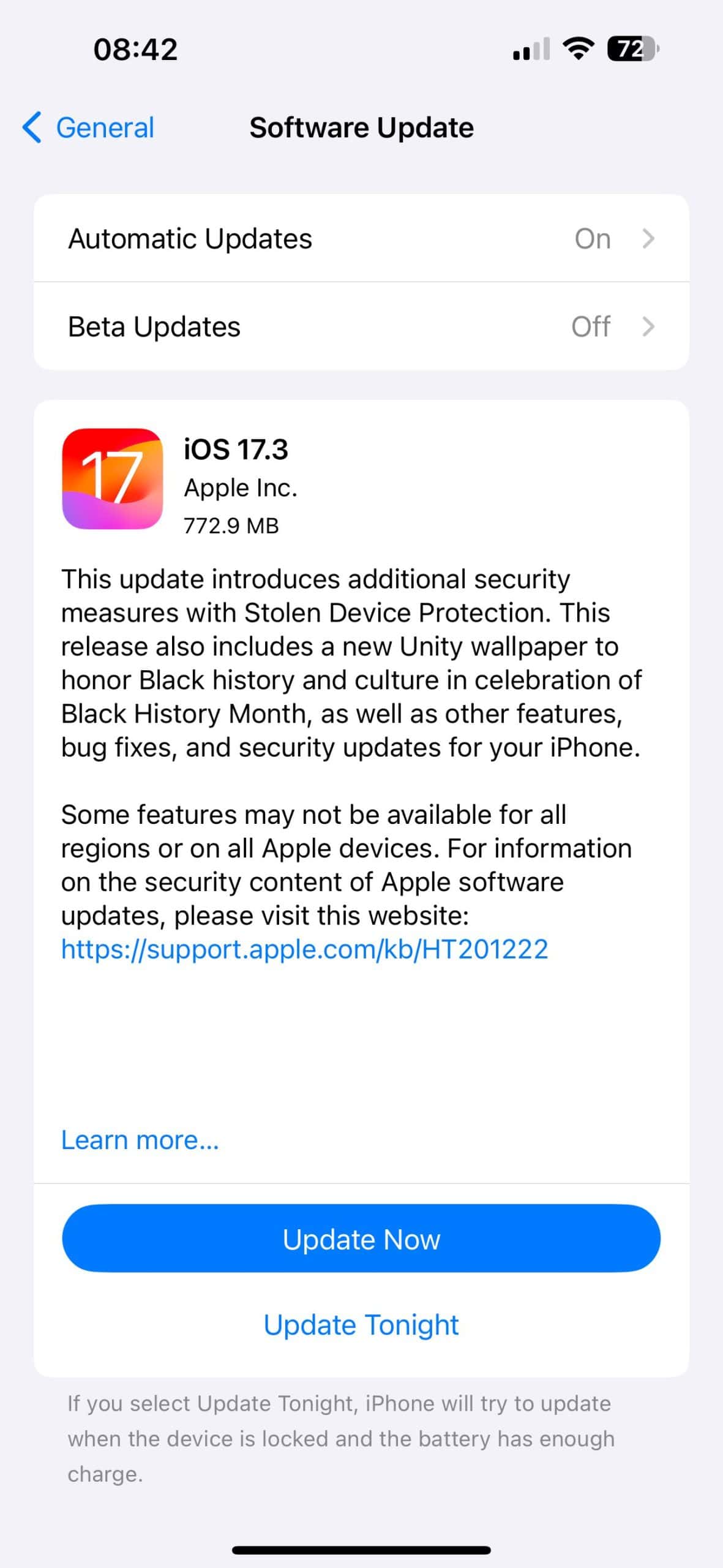A detailed and cleaned-up descriptive caption for the image:

The image displays a software update screen on an Apple iPhone with a grey background. At the top center, it prominently reads "Software Update," while in the upper left corner, "General" is displayed in light blue with a left-pointing arrow beside it. Below the "Software Update" heading, two selection boxes are visible: "Automatic Updates" set to On and "Beta Updates" set to Off.

Further down, a large white box contains the details of the latest software update. On the left side of this box is a thumbnail marked with the number 17. To the right, the text specifies the update as "iOS 17.3" by "Apple Inc." with a file size of 772.9 MB. The update description mentions introducing additional security measures with stolen device protection, a new Unity wallpaper to honor Black History and Culture for Black History Month, and other features, bug fixes, and security updates. It notes that some features may not be available in all regions or on all Apple devices. A hyperlink is provided for more information on the security content of Apple software updates.

At the bottom left of the text box, there is a "Learn More" link. Centered at the very bottom is a blue-highlighted button labeled "Update Now," with a blue-hyperlinked option below it stating "Update Tonight."